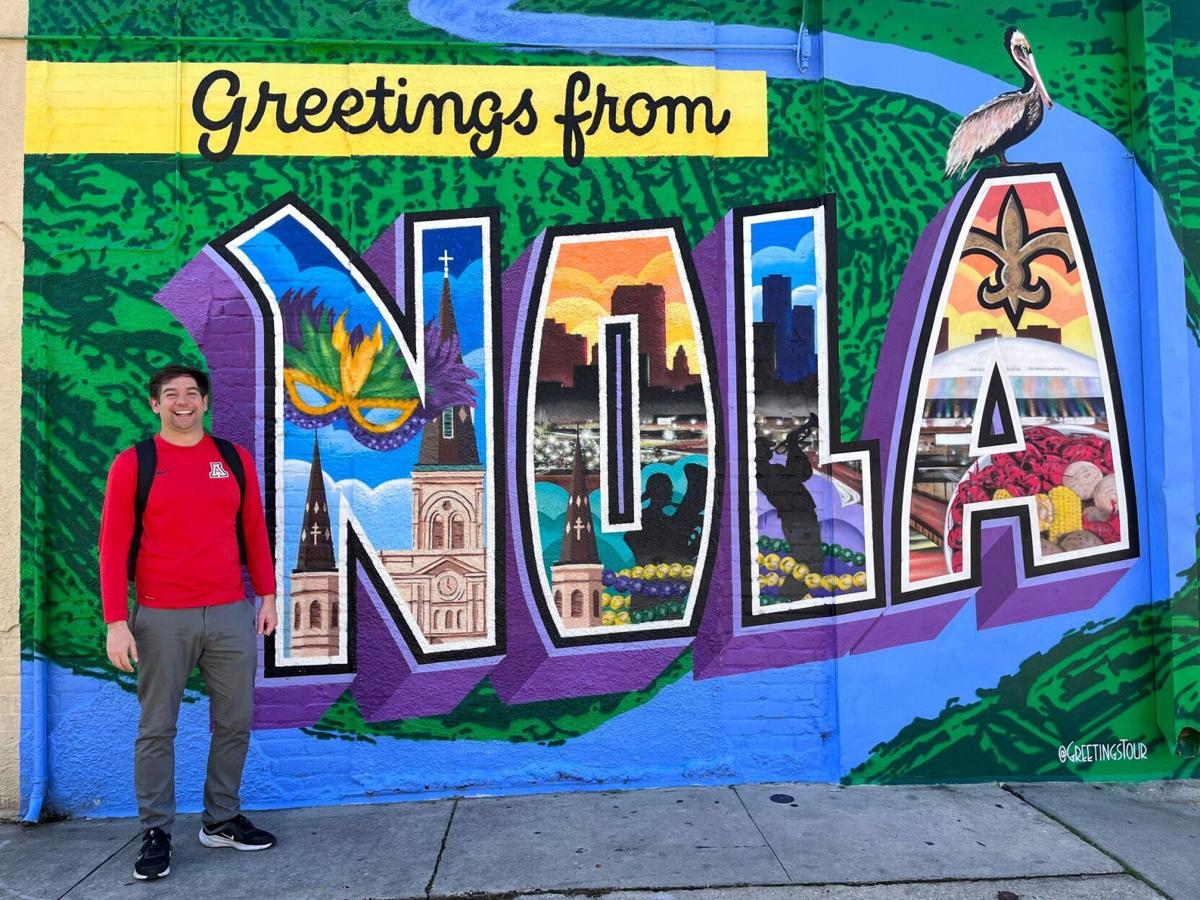In an outdoor daytime photograph, a rectangular image about six inches wide and four inches high captures a vibrant scene. In the bottom left-hand corner, a cement sidewalk extends up about half an inch and goes over three-quarters of an inch to the right. Standing on the left-hand side of the sidewalk is a laughing man of Caucasian descent with brown hair, eyes locked on the camera. He is dressed in a long-sleeve red shirt, gray pants, and black shoes, with the straps of a black backpack visible around his shoulders. 

The man stands against a wall adorned with a colorful mural. The wall’s original light gray stone is partially visible on the left, but the mural covers the majority of it. From the upper left toward the right, a green, grassy area transitions into a blue river, with more greenery on the upper and lower right corners. A yellow banner emerges from the upper left, bearing the black cursive text, "Greetings From." Below this, large raised letters spell out "NOLA," each filled with distinctive images. 

The "N" features a Mardi Gras mask and what appears to be a church. The "O" includes the top of a spired church against a city skyline at dusk. The "L" showcases a jazz musician playing a trumpet, and the "A" is decorated with a fleur-de-lis and a domed building, topped with a perched pelican. Enhanced with a purple shadow effect, the letters give the mural a dynamic, raised appearance. In the lower right corner of the mural, the phrase "Greetings Tour" or "At Greetings Tour" is painted in white, further emphasizing the festive atmosphere of New Orleans.